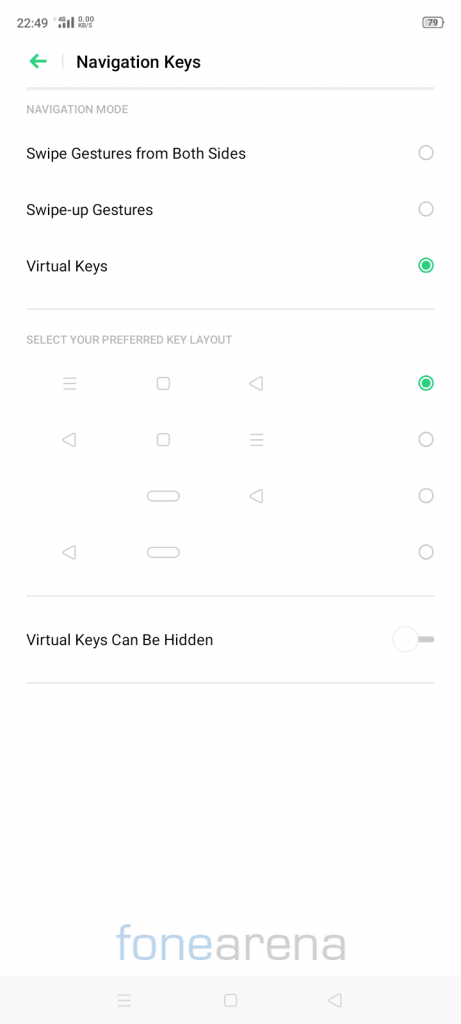A detailed screenshot of a smartphone settings page is depicted in the image. At the top left, the time is displayed as 22:49, next to the signal bars and another indiscernible icon. The user is navigating through settings specifically related to system navigation options. The options presented include "Navigation Keys," "Swipe Gesture from Both Sides," "Swipe Gesture," "Swipe Up Gestures," and "Virtual Keys."

The user has selected "Virtual Keys" and chosen the first key layout option, which arranges the keys with the 'Tab' screen on the far left, 'Home' in the center, and 'Back' on the far right. Additionally, a setting option stating "Virtual key can be hidden" is visible above these choices. At the bottom of the screen, there are buttons for navigation, including the 'Back,' 'Tabs,' and 'Home' icons recognizable on most smartphones.